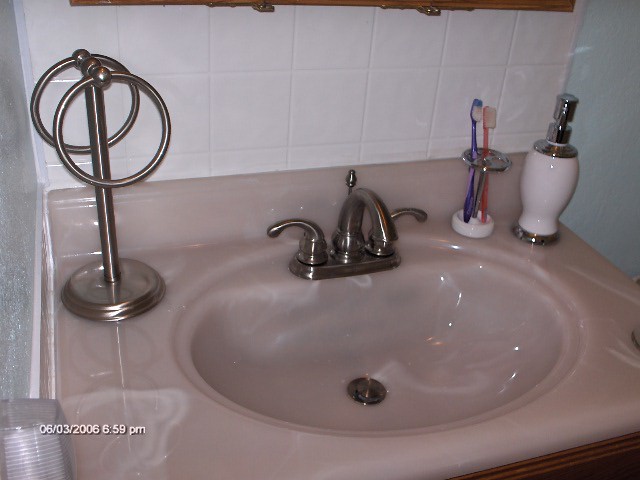The image depicts a pristine pink-hued sink with a sophisticated faucet featuring two handles, presumably for hot and cold water. The sink gleams with cleanliness and meticulous care. To the right of the faucet are two toothbrushes; one purple and one red, both with transparent handles, adding a touch of color to the setting. Adjacent to the toothbrushes is an elegant white hand wash dispenser adorned with a metallic silver release button, hinting at modern convenience. The backdrop consists of neat white square tiles that accentuate the sink's color. The surrounding wall has a subtle blue tinge, providing a gentle contrast. Above the setup is a wooden mahogany cabinet, partially visible but sharply cut off at the top in the image. To the far left, a towel holder with two empty circular rings suggests the towels are currently being laundered.